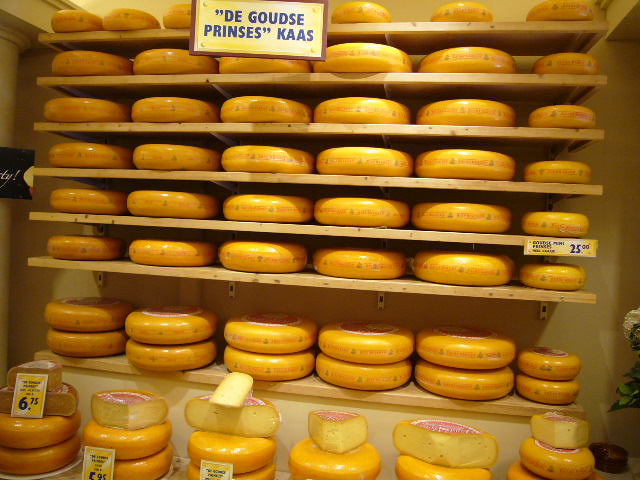The photo captures a neatly arranged wall display of cheese wheels, set on six evenly spaced wooden shelves. Each shelf holds circular, yellow wax-coated cheese wheels, all of the same variety but varying in shape, thickness, and size. At the top of the display, there is a sign in French that reads 'Des Gouttes Princesses,' while another version of the sign, possibly 'Die Gütze Prinzess Kass' or 'Degoutes Princesse Kaz,' also appears. Price tags on the shelves indicate some cheese is priced at $25 and $6, though the currency is not specified. In the foreground, there are slices and wedges of the cheese arranged to showcase the interior.